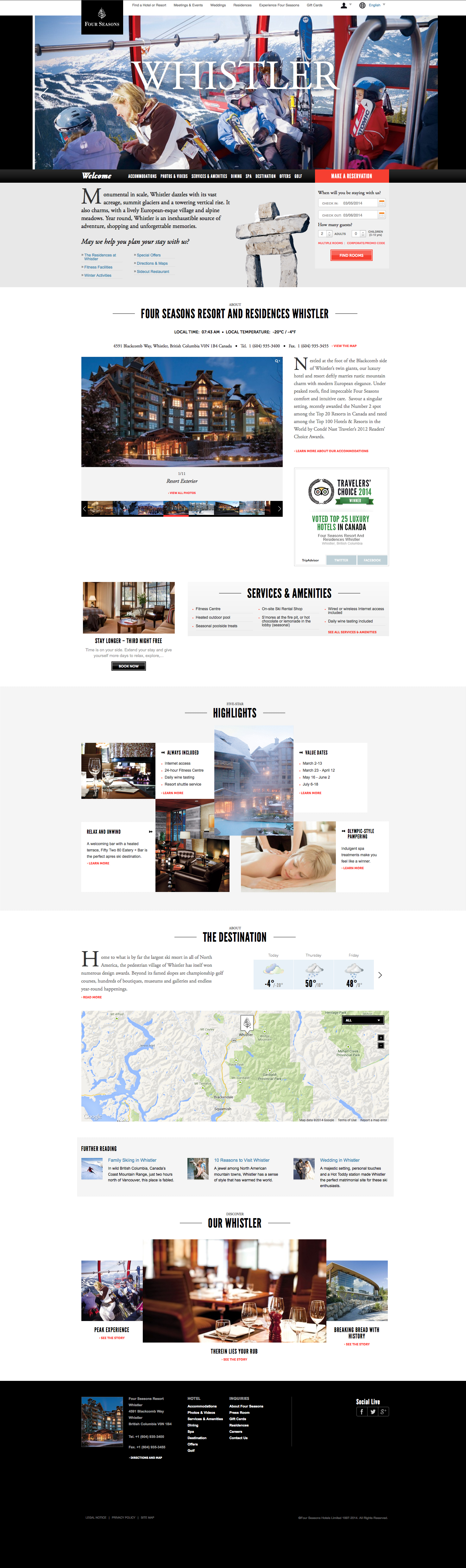This image captures the entire front page of the website for Whistler, a renowned destination in British Columbia, presented in a long, portrait-style format. At the very top, there is a background image featuring people on a ski lift, with one individual holding a snowboard, indicating they are ascending a skiing mountain. The page is introduced with a caption that reads:

"Monumental in scale, Whistler dazzles with its vast acreage, summit glaciers, and towering vertical rise. It also charms with a lively European-esque village and alpine meadows. Year-round, Whistler is an inexhaustible source of adventure, shopping, and unforgettable memories."

Below this introductory text, there is an option to make a reservation, allowing users to input check-in and check-out dates, select the number of guests, and search for available rooms. The website highlights the Four Seasons Resort and Residences as a prominent accommodation option, displaying various images of the resort.

Detailed information about the Four Seasons Resort and Residences is provided, including its location in Whistler, British Columbia, along with its contact phone number. The highlights section outlines the value dates and amenities that are always included, such as internet access, a 24-hour fitness center, and daily wine tastings.

Further down, a map of the Whistler area is displayed, accompanied by a weather forecast for the upcoming days. The forecast ranges from -4 degrees to 50 degrees over three days (Tuesday to Thursday), with options to view the weather for today, Wednesday, Thursday, and Friday.